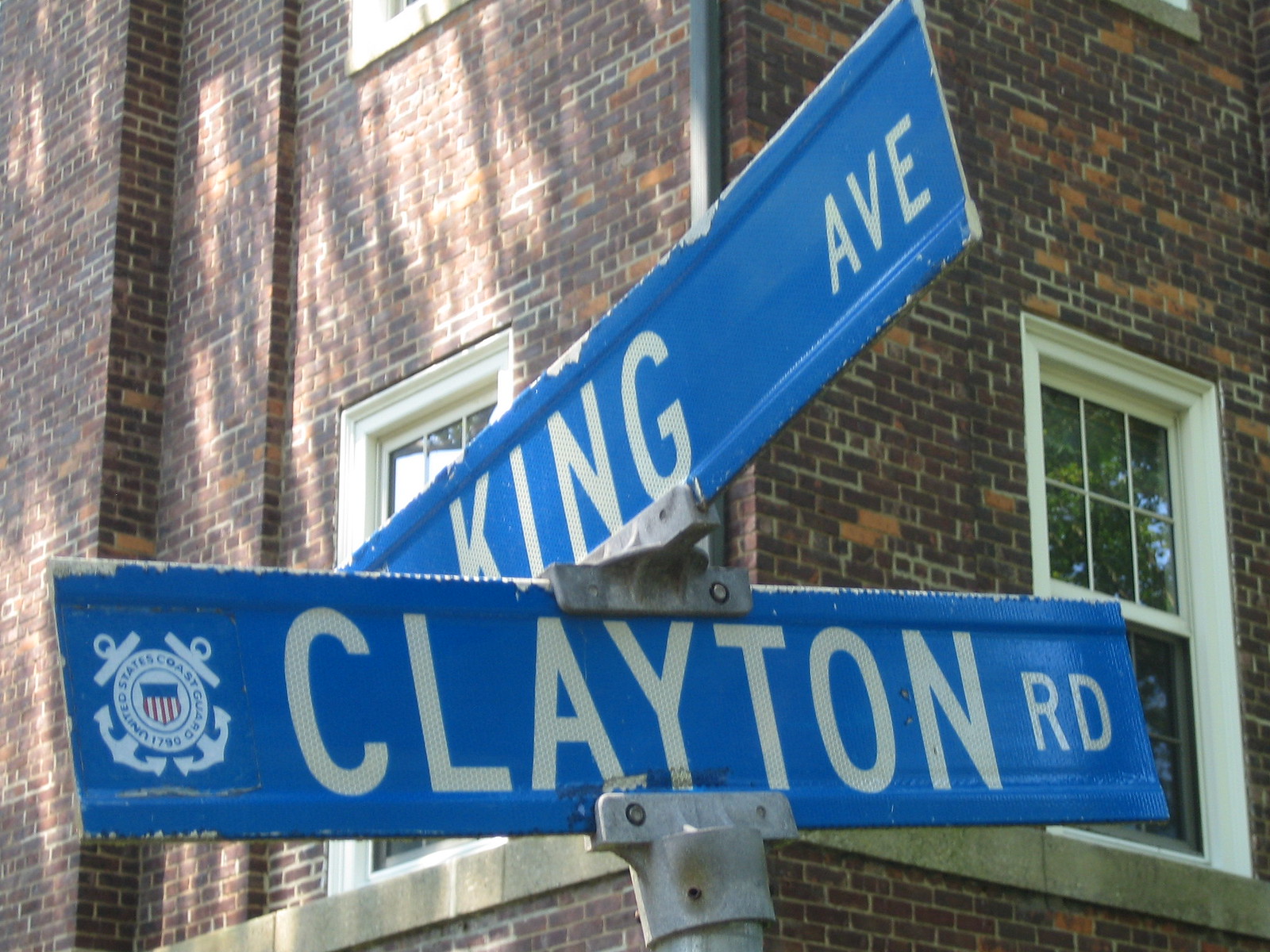In this photograph, the primary focus is on two intersecting street signs set against the backdrop of a multi-story brick building. The building occupies the entire background of the image, though only a small section of it is visible. Notably, the building appears to have several stories; clearly visible are two windows on what seems to be the second story, while the bottom corners of a couple more windows can be seen on the third story. The windows feature a white trim and are designed with a six-over-one pane configuration.

Dominating the scene, the street signs are a vivid blue with white text. One sign reads "King Avenue" and the other "Clayton Road." Both signs are mounted together on a single metal pole, joined by a metal bracket. This carefully arranged setup ensures that each street name is easily readable from different directions.